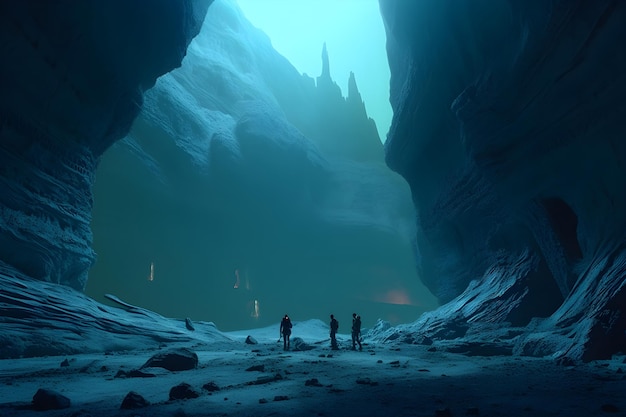The image depicts a vast, rocky cavern with towering walls that curve slightly inward, bathed in a blue hue. The base of the cavern is strewn with a variety of jagged rocks and loose dirt, capturing a rugged terrain. In the foreground, there are three small figures, their black outlines suggesting they're clad in some form of gear that could be mistaken for spacesuits or hiking gear. They appear to be handling weapons and are positioned roughly an inch from the bottom of the image, with one figure on the left walking away from the cave. The other two figures are facing to the left, standing close together. The cavern stretches far into the distance, and the scene is illuminated by a faint bluish sky visible through a narrow opening far above. In the background, near the base of the cavern walls, a set of four white lights can be seen, adding a touch of mystery and possibly hinting at some form of hidden technology. Overall, the image exudes a sci-fi ambiance, blending elements of natural cave formations with a futuristic, otherworldly atmosphere.